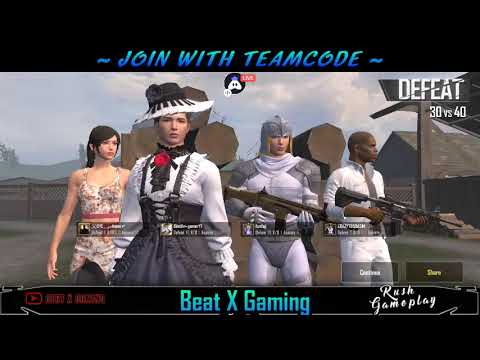In this computer-generated game screenshot, we see an image framed by a black border with the phrases "Join with Team Code" in blue at the top and "Beat X Gaming Rush Gameplay" along with "Defeat 30 vs 40" at the bottom. At the center of the image stand four characters. On the left, a woman with black hair tied up is dressed in a four-row strapped tank top paired with a skirt. Beside her, another woman is attired in a black and white Victorian-style dress, accented with a tall hat and a red flower on her chest. To the right of the women, two men in futuristic white and gray uniforms are holding long guns. The man immediately to the right of the women is in a gray helmet and white pants, aiming his gun to the left. The man at the far right also wears white pants and carries his gun pointed to the right. The background features a concrete setting with a fence and a few buildings, suggesting an urban environment. The image predominantly displays colors like black, white, blue, gray, red, and tan.